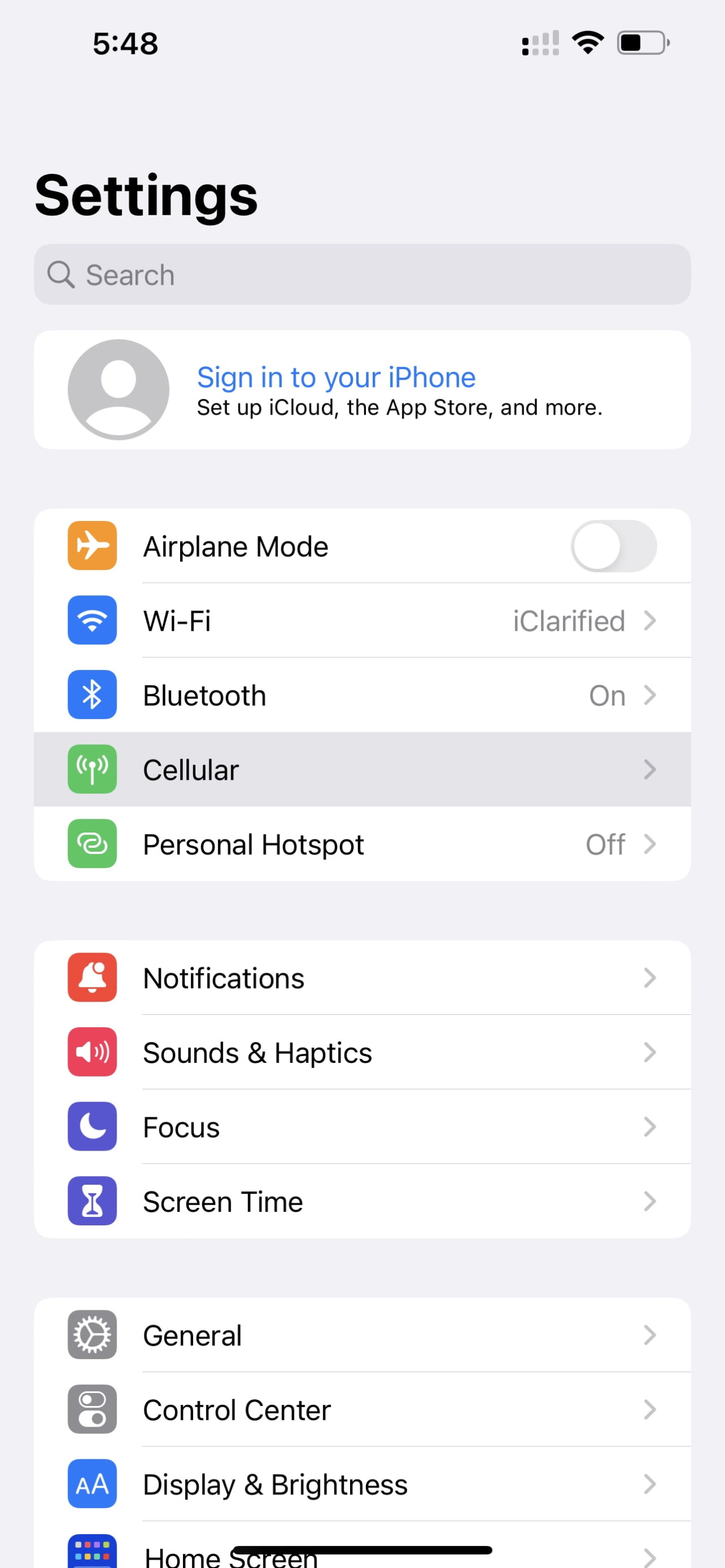This image is a detailed screenshot of the settings menu on an iPhone, captured from a mobile device. At the top left of the screen, the time is displayed as 5:48. Adjacent to the time, the cell reception icon shows one out of five bars, indicating weak signal strength. Next to that, the Wi-Fi icon is fully illuminated, indicating a strong Wi-Fi connection. The battery icon shows approximately 50% charge remaining.

Below the status indicators, the word "Settings" is prominently displayed in large black text. Directly beneath this header is a search bar stretching across the entire width of the screen, featuring a magnifying glass icon and the placeholder text, "Search."

Following the search bar, there is a white bar containing a blank profile picture icon and the text, "Sign in to your iPhone. Set up iCloud, the App Store, and more." This is an invitation to the user to log in to their Apple ID for accessing various services.

The main list of settings begins with the following items, each accompanied by an icon on their left:
1. **Airplane Mode** (currently toggled off)
2. **Wi-Fi**
3. **Bluetooth**
4. **Cellular**
5. **Personal Hotspot**

A slight space separates this group from the next set of settings, which includes:
1. **Notifications**
2. **Sounds & Haptics**
3. **Focus**
4. **Screen Time**

Another small space precedes the final group in this view, which comprises:
1. **General**
2. **Control Center**
3. **Display & Brightness**
4. **Home Screen**

Each of these sections is clearly delineated and includes a corresponding icon for easy identification. The overall layout is clean, organized, and user-friendly.